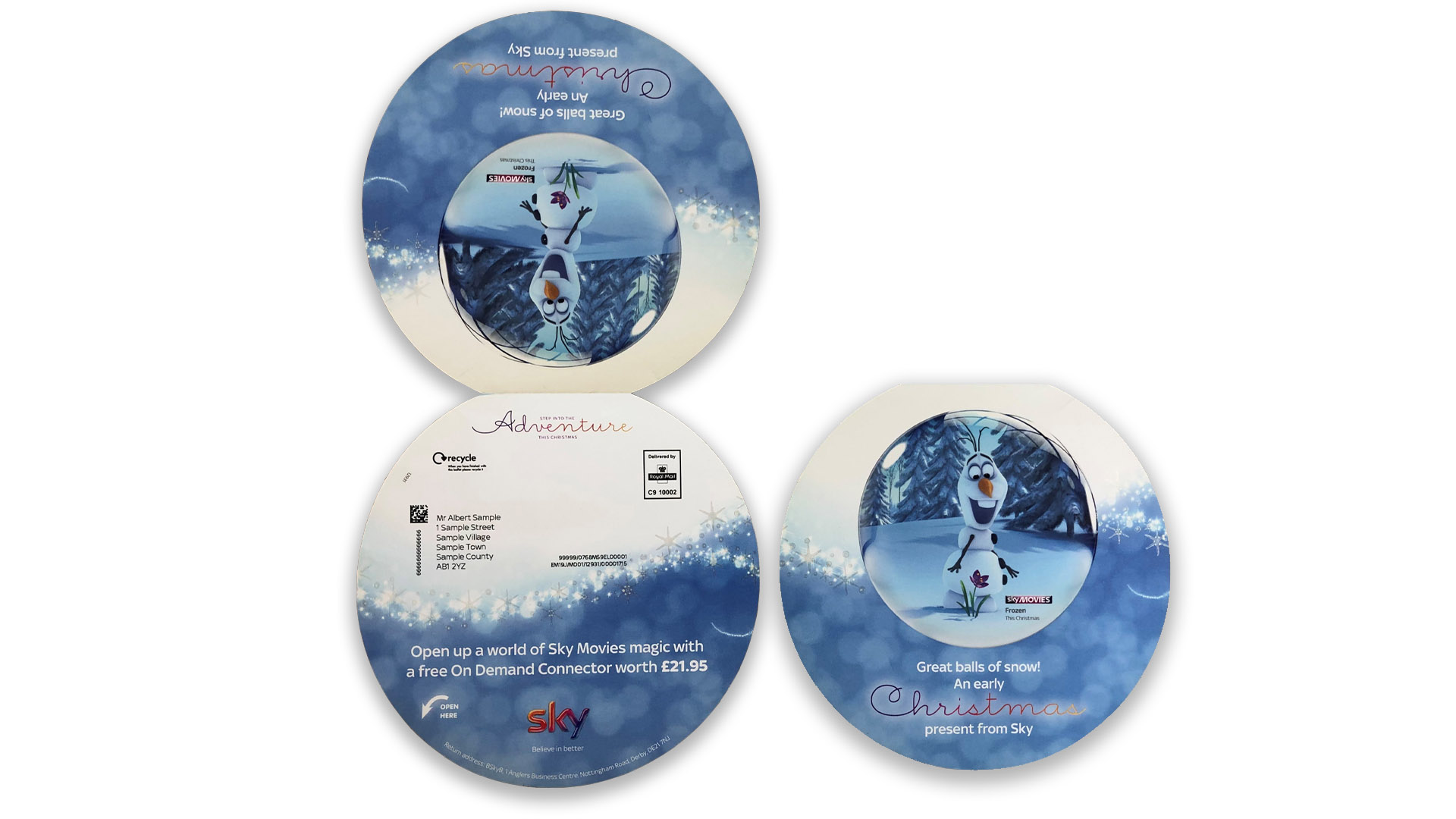The image showcases a promotional booklet related to the movie "Frozen," featuring Olaf the snowman. The booklet is divided into three circular sections. The top left and bottom right circles display an image of Olaf, the snowman from "Frozen," set against a blue and white snowy ice theme. The bottom right circle includes text in white that reads, "Great Balls of Snow, an early Christmas present from Sky." The "Christmas" text is in red and cursive. The bottom left circle is split into two halves: the top half is white, and the bottom half is blue. Wavy white bubbles separate the two halves. The top portion features the word "ADVENTURE" in red, while the bottom blue section contains white text that states, "Open up a world of Sky movie magic with a free On Demand connector worth £21.95." Overall, the booklet's back cover emphasizes the adventure theme, surrounded by a wintry, sparkly design, enhancing the magical and festive appeal.